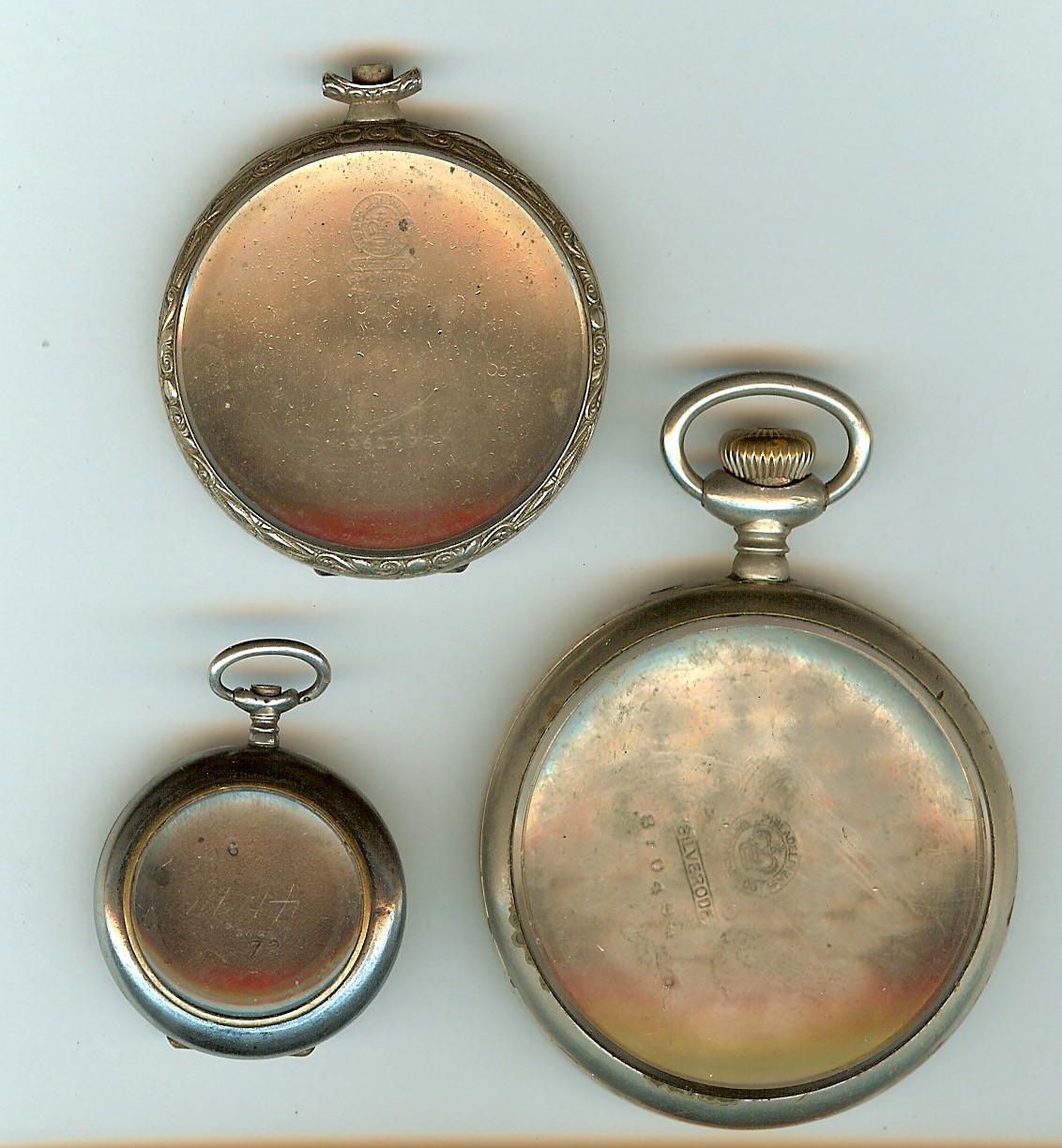This photograph features three antique pocket watches set against a grayish-white background. The watches, reminiscent of the timepieces traditionally carried in suit coat pockets on chains, vary in size and detailing. The watch in the upper left corner is a medium-sized, circular piece with a clasp at the top. It has intricate rope-like detailing around the edge and exhibits a patina, suggesting age, though the embossed image in the center remains indistinguishable. Below it, in the bottom left, is the smallest watch, also circular with a clasp, and displays a similar patina with an unreadable etching on its back. This smaller watch has a slightly silver hue, particularly around the clasp. The largest watch is situated to the right. It too is circular, with a top clasp. Its back is relatively plain, marked only by signs of rust around the edges and indistinguishable lettering or designs. All three watches, shown from the back, hint at maker’s marks that are too minute to discern without magnification.